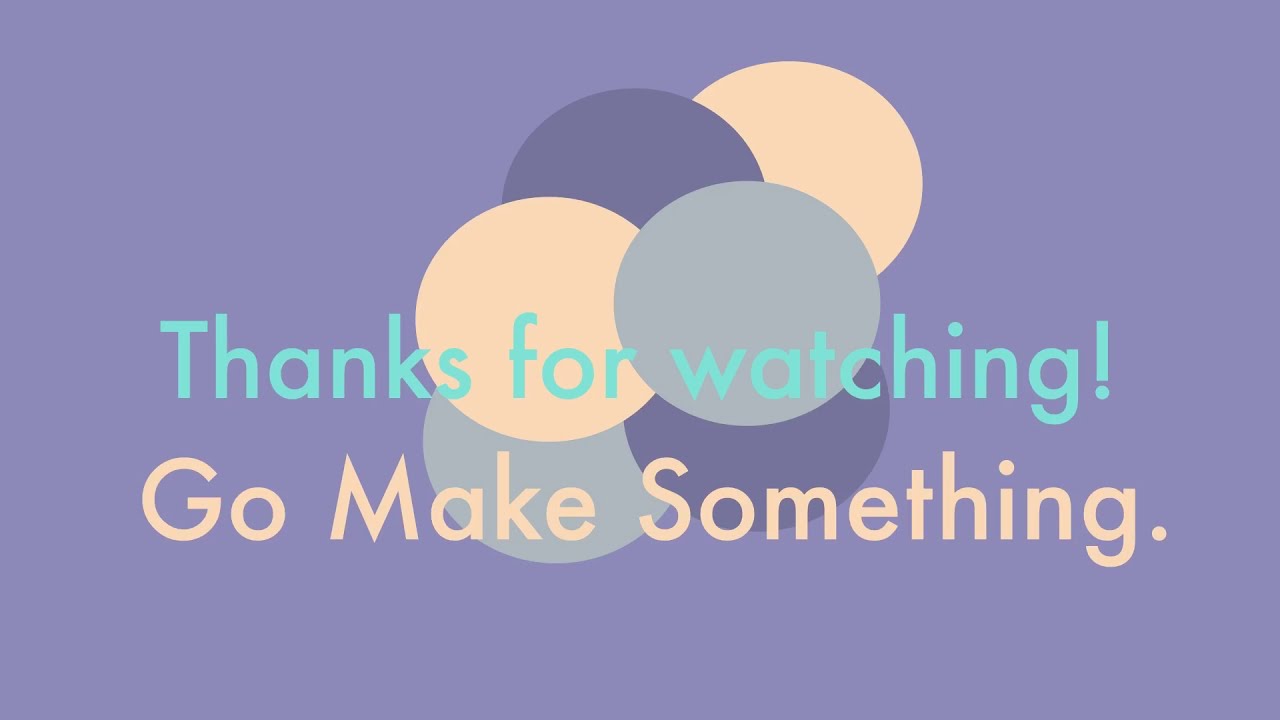The image features a soft, pastel lilac background with two lines of text centrally positioned over an intricate graphical design composed of six overlapping circles. The top line of text, written in a vibrant light blue color, reads "Thanks for watching!" followed by an exclamation mark. Directly beneath it, in a pale peachy tan color, are the words "Go make something." Behind these lines, six interconnected circles are arranged with two in dark bluish-purple, two in pastel yellow, and two in gray. The circles are clustered toward the center and upper right-hand side of the image, adding a playful yet orderly touch to the design.